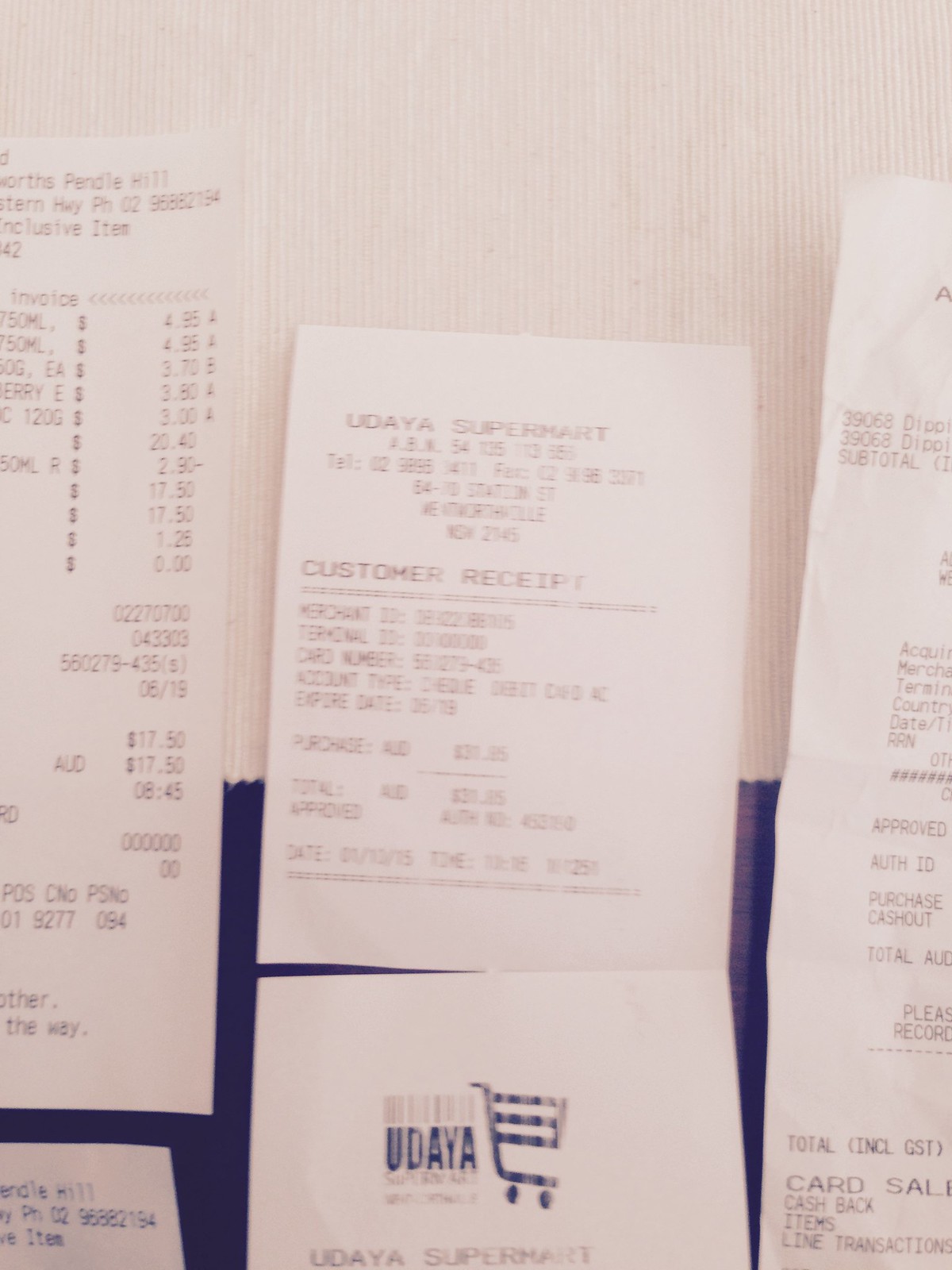The photograph captures a disorganized array of several white receipts, possibly five or six, layered one in front of the other. Some receipts are partially cut off due to the framing of the image. Among the visible details, one receipt prominently features a black silhouette line drawing of a shopping cart alongside the name "Udaya," indicating it is from a supermarket. These receipts are printed with black text and include various logos and icons. The background consists of a two-toned tablecloth, white at the top and transitioning to dark blue at the bottom. The image appears slightly blurry, perhaps suggesting a hasty capture.